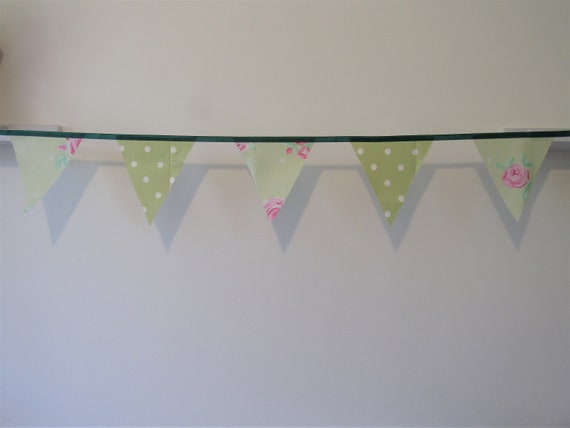This photograph, taken indoors, features a decorative party banner showcasing five upside-down triangular pennants strung along a dark green line. The wall in the background is light gray, and the banner casts a shadow on it. The banner runs horizontally across the wall from the upper left to the upper right, about an inch from the top. 

The triangles are alternately patterned: three of them have a light green or grayish background adorned with pink flowers and green leaves, while the other two pennants feature a darker, moss-green color with white polka dots. The delicate design captures a whimsical and festive atmosphere, ideal for a display picture, perhaps showcasing a product for sale online.